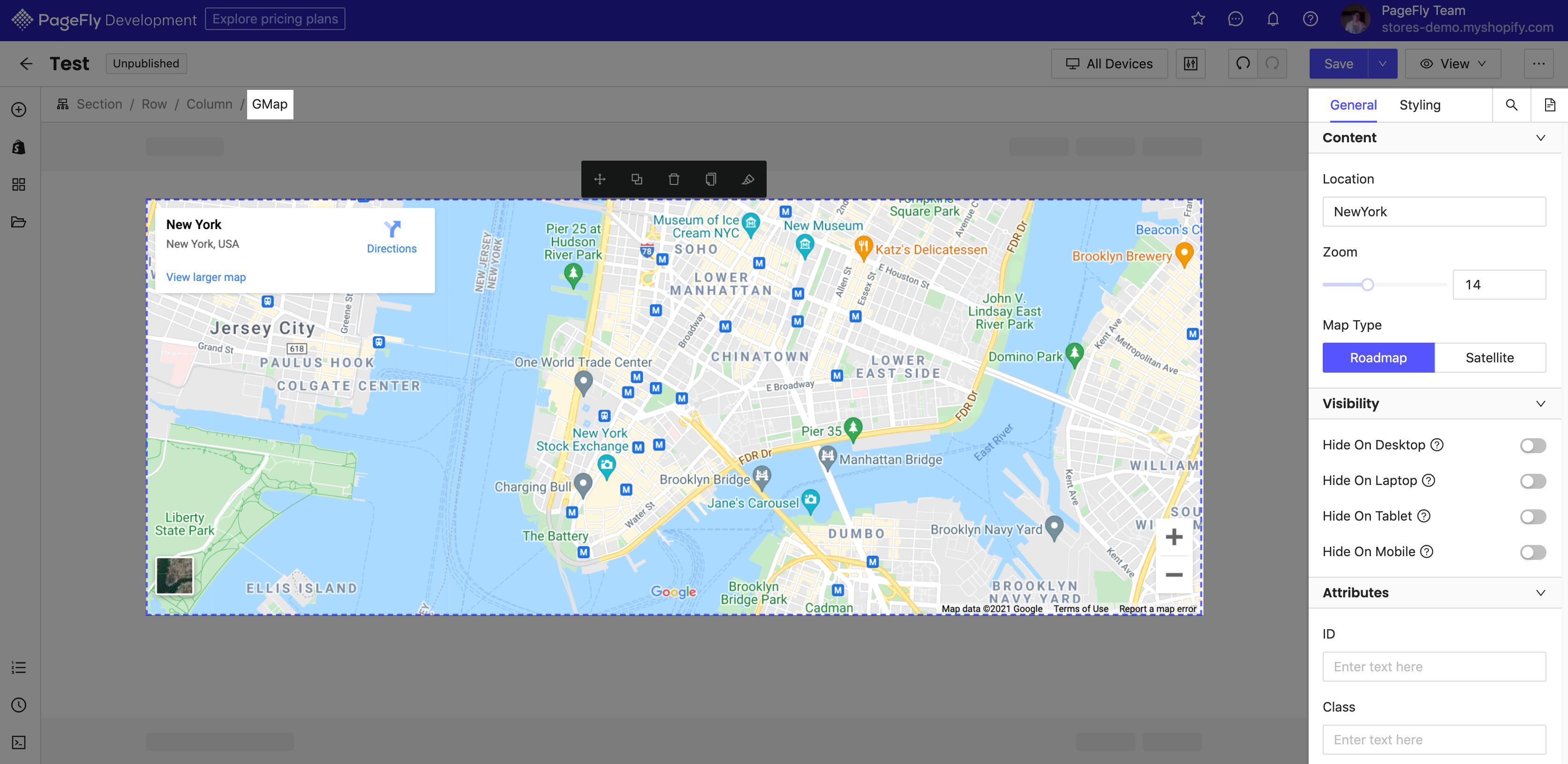The image is a detailed screenshot of a web page under a gray overlay titled "PageFly Development," with the page focusing on exploring pricing plans. However, the focal point of this screenshot is an overlaid map centered on New York, New York, USA. The map prominently displays several points of interest, each identified with various colored pins.

Significant landmarks and locations such as Jersey City, Lower Manhattan, Domino Park, Brooklyn Navy Yard, Ellis Island, New York Stock Exchange, Charging Bull, and One World Trade Center are labeled. Notably, Katz's Delicatessen is marked with an orange pin featuring a fork and knife icon, while Pier 25 at Hudson River Park is marked with a green pin. Scattered throughout the map are small squares with blue backgrounds showcasing the letter "M," indicative of specific points that require attention.

To the right of the map is a settings panel under a highlighted tab labeled "General" with adjacent options for "Styling" and "Content." Within the "General" settings, the location is set to New York with a zoom level of 14. The map type is selected as "Road Map," contrasting the alternative "Satellite" view. Visibility settings for different devices (Desktop, Laptop, Tablet, Mobile) are displayed but are all currently disabled, meaning the map is visible on all devices.

Overall, the map overlay dominates the screenshot, providing a detailed view of various New York points of interest along with customizable settings for display preferences.